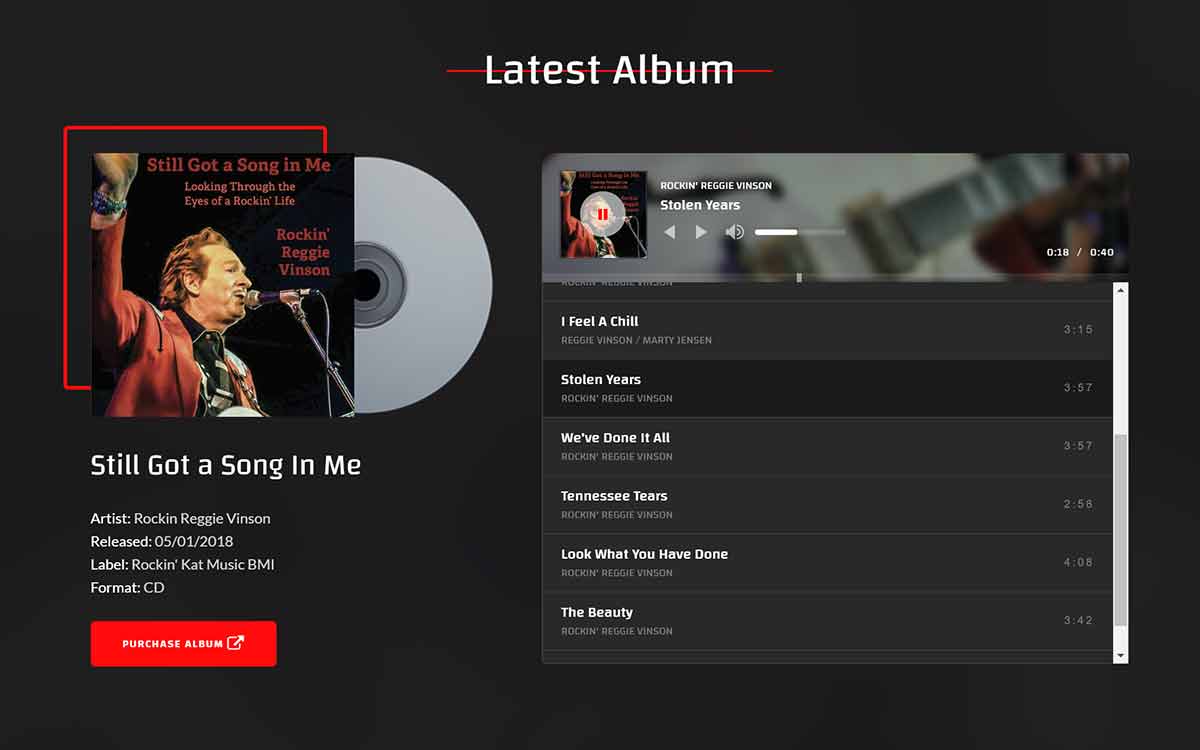This is a detailed screenshot from an unknown source featuring promotional content for the latest album by Rockin' Reggie Vinson. The background is black, giving prominence to the elements on the screen. At the top, the words "Latest Album" are displayed with a thin red horizontal line running behind them.

To the left, the album cover art showcases a middle-aged man, presumably Rockin' Reggie Vinson, wearing a red suit jacket. He has his right hand raised in the air, adorned with several bracelets or similar items around his wrist, and is enthusiastically singing into a microphone on a stand. The album title, "Still Got a Song in Me: Looking Through the Eyes of a Rockin' Life," is prominently displayed along with the artist's name, Rockin' Reggie Vinson.

The cover also includes an image of a CD emerging from it, with additional album details provided below:
- Title: Still Got a Song in Me
- Artist: Rockin' Reggie Vinson
- Released: 05-01-2018
- Label: Rockin' Cat Music BMI (spelled as K-A-T)
- Format: CD

At the bottom, a red rectangle indicates a call-to-action button labeled "Purchase Album."

On the right-hand side of the screen, the current track "Stolen Years" is 18 seconds into its 40-second playtime. Below, the tracklist is provided with detailed information including titles, contributing artists, and durations:
1. "I Feel a Chill" - Reggie Vinson, Marty Jensen (3 minutes 15 seconds)
2. "Stolen Years" - Rockin' Reggie Vinson (3 minutes 57 seconds)
3. "We've Done It All" - Rockin' Reggie Vinson (3 minutes 57 seconds)
4. "Tennessee Tears" (2 minutes 56 seconds)
5. "Look What You Have Done" - Rockin' Reggie Vinson (4 minutes 8 seconds)
6. "The Beauty" - Rockin' Reggie Vinson (3 minutes 42 seconds)

This caption provides a comprehensive and detailed overview of the screenshot, conveying all relevant information about the album and its features.